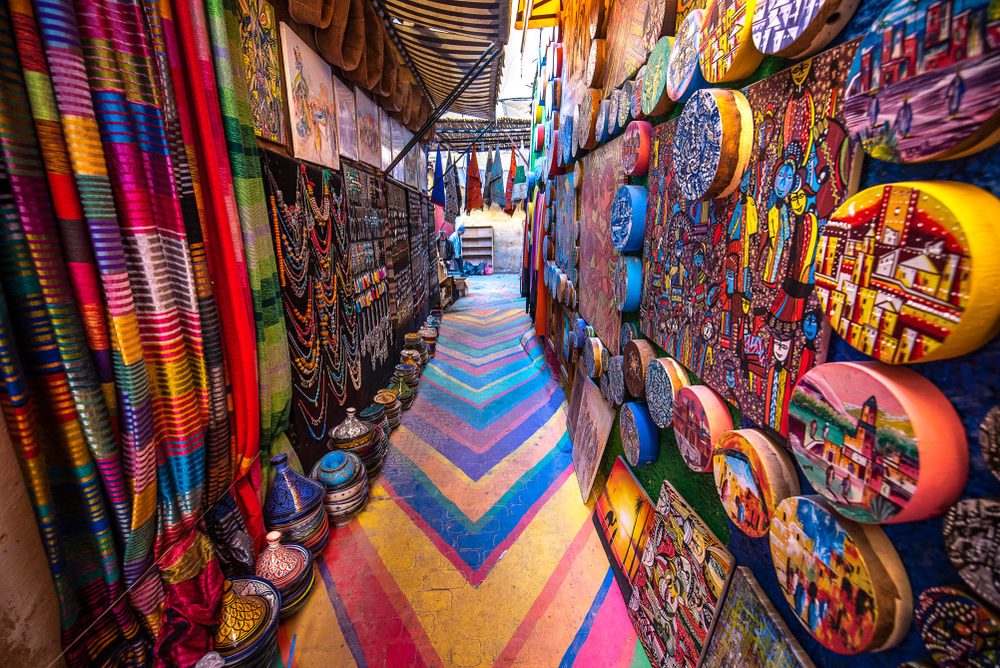The photo captures a bustling outdoor marketplace, possibly situated in India, the Middle East, or Africa, brimming with vibrant Eastern aesthetics. On the left, a rich display of ornate necklaces, intricately decorated vases, water pots, and a variety of colorful carpets draws attention. The right side features an array of round, vividly colored paintings showcasing diverse artistic styles, from symmetrical and hyper-realistic to abstract. Dominating the walkway is a striking chevron pattern in an array of rainbow colors, adding to the lively atmosphere. Further enriching this eclectic scene are silk robes, clay pots, and vivid fabrics. The marketplace is an explosion of colors and textures, reminiscent of a traditional bazaar, with tents and stalls offering jewelry, talismans, scarves, and more. This vibrant setting weaves together a tapestry of cultural artistry and warmth, inviting onlookers to explore its myriad treasures.